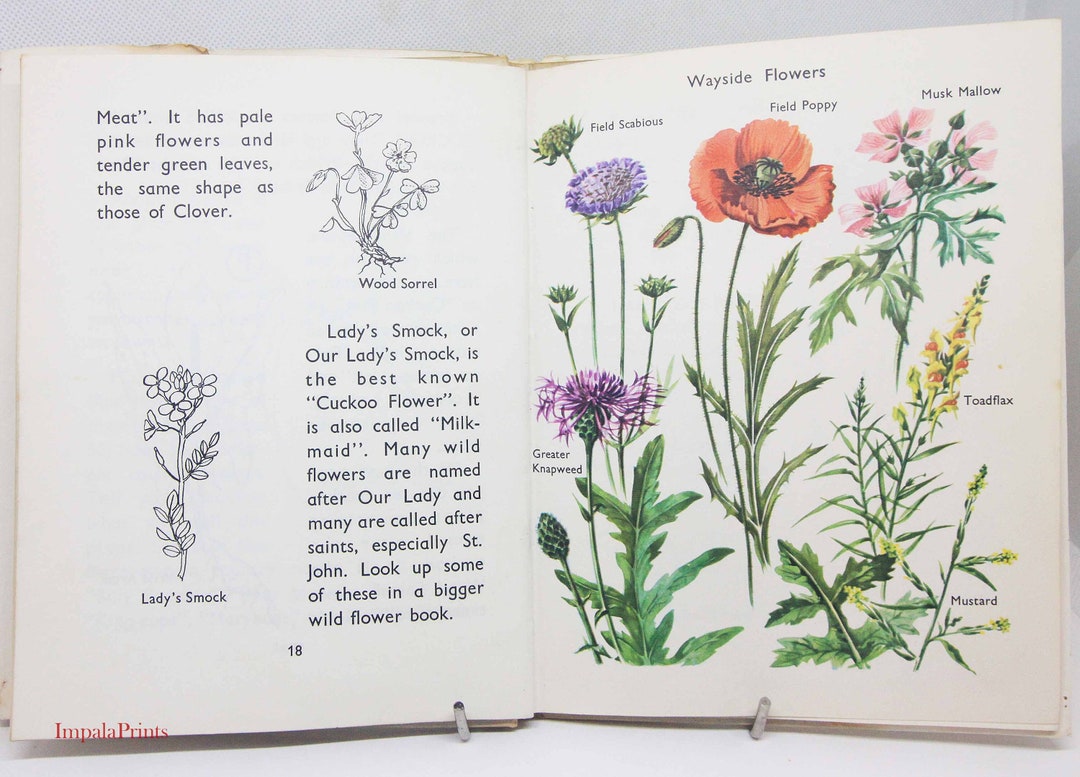This image captures an open spread of a botanical book titled "Impala Prints." On the left-hand page, detailed black and white illustrations and text describe two plants. The page opens with the word "Meet" accompanied by a drawing of a pale pink flower with tender green leaves shaped like clovers, identified as Wood Sorrel. Below, there is another illustration labeled Lady Smock, with descriptive text highlighting that Lady Smock, also known as Cuckoo Flower or Milkmaid, is one of many wildflowers named after religious figures like Our Lady and various saints, especially St. John. Readers are encouraged to look up similar flora in a more extensive wildflower book. The page is marked with the number 18 at the bottom left corner. Contrasting this, the right-hand page features vibrant watercolor images of several wildflowers labeled as Wayside Flowers. These include the purple Field Scabious and Greater Knapweed, the orange Field Poppy, the pink Musk Mallow, and the yellow Toadflax. The background of the book is white, emphasizing the colored illustrations on the right.